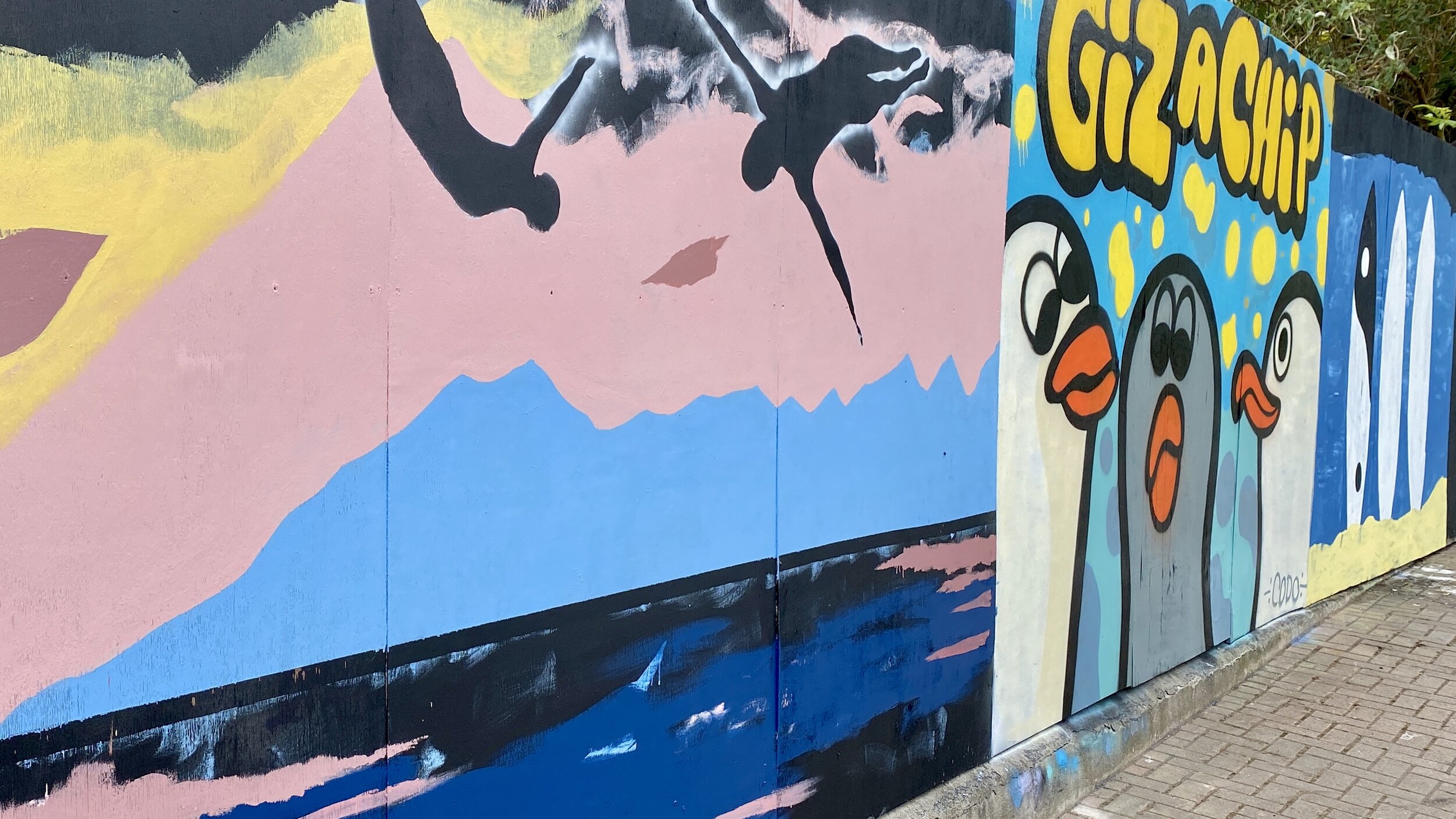This photograph captures a colorful outdoor mural spanning the width of a wooden wall, set against a slightly cloudy sky. The mural exhibits distinct sections of street art, beginning on the left with an abstract painting in shades of light blue and coral, transitioning towards the middle where two black silhouette figures dive into a vibrant blue ocean under a dynamic sky of blue and white. Adjacent to this, the central section features three cartoonish, penguin-like figures—two white with orange beaks and one purple, also with an orange beak—accompanied by bold yellow text reading "Giz a Chip," outlined in black. On the far right, the mural showcases three artistically-rendered, cartoonish surfboards leaning against a backdrop suggestive of a sandy beach scene, all depicted in loose, vibrant strokes. The mural is set above a stone walkway, emphasizing the artwork's placement in an urban outdoor setting devoid of people or additional text, effectively highlighting the mural's vivid and playful aesthetic.